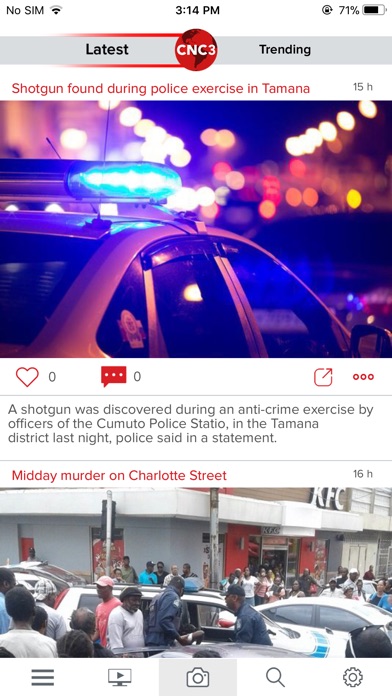This phone screenshot captures a typical news feed interface complete with the standard phone status ribbons at the top and bottom, displaying various cell phone icons. Dominating the center area is a circular logo at the top, labeled "CNC3," flanked by tabs reading "Latest" on the left and "Trending" on the right, suggesting that this is a news app.

The first news headline, in red text, reads: "Shotgun found during police exercise in Tamana." Below it is a stock image featuring a police car parked on a street, used to represent the news article. The brief description that follows states: "A shotgun was discovered during an anti-crime exercise by the officers of the Komodo Police Centennial in Tamana district last night, police said in a statement." This article was posted 15 hours ago.

The next article headline reads: "Midday murder in Charlotte Street," accompanied by a photograph showing a crowd, mostly African-American individuals, gathered on a street lined with police cars. In the background to the right, a KFC restaurant is visible, indicating the real-life location of the incident. This news article was posted 16 hours ago.

Overall, the screenshot effectively showcases a selection of recent news articles curated in the "Latest" section of this news app.